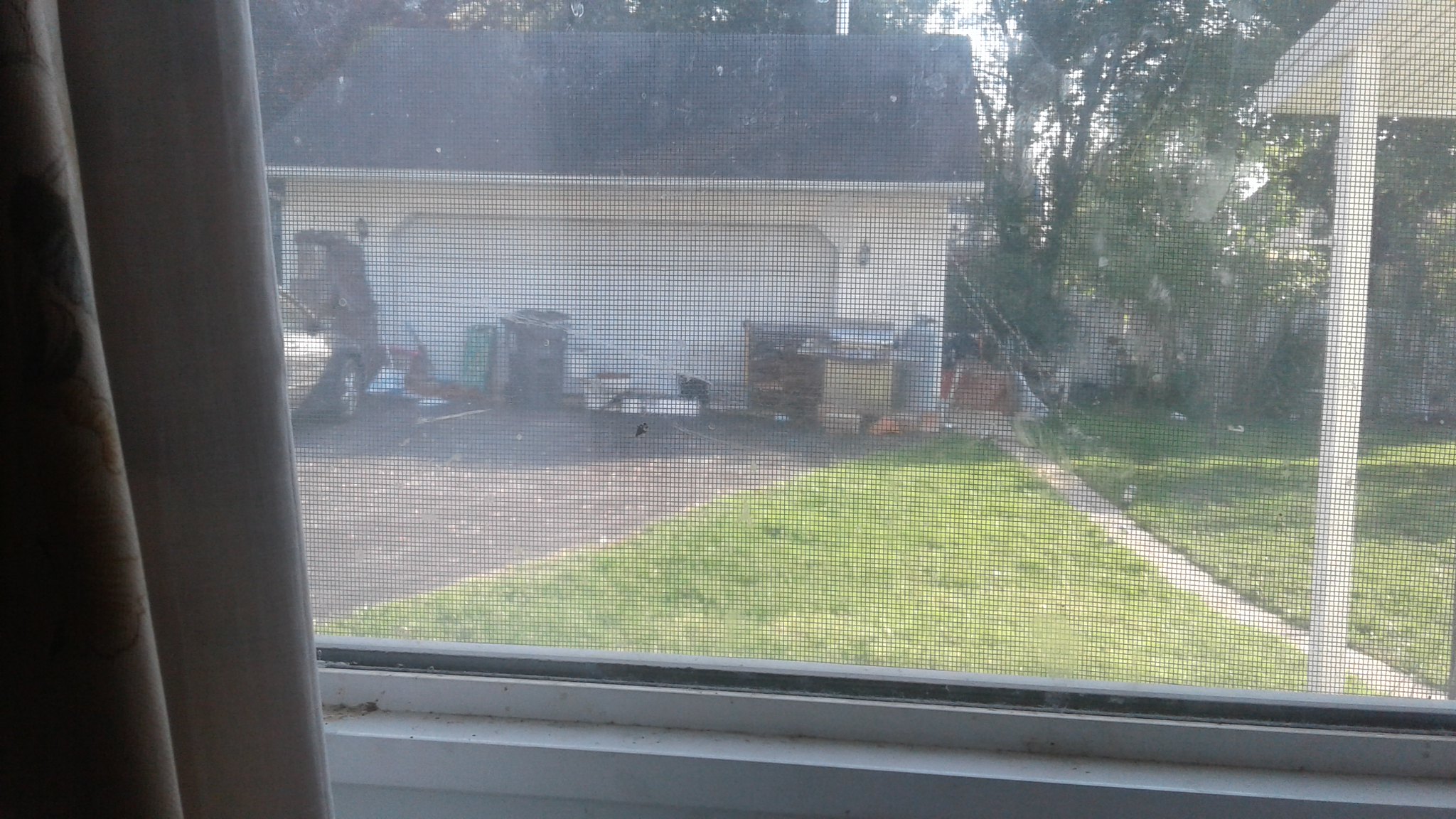The photograph captures a scene through a mesh screen or window, creating a slightly fuzzy effect. Taken from inside a house, the view encompasses a garage area with a mix of detailed elements. In the foreground, a white patio roof frames the scene with brown curtains and a dirty windowsill to the right. The garage, prominently beige or pale cream in color, features a white double door with a black, book-orientated roof. Scattered across the black driveway and gray walkway are various items: boxes, a wheelie bin, a tall gas bottle, fishing poles, and what appears to be a desk or cabinet with drawers, hinting at possible recent moving activity. The left side of the image reveals the front end of a car, while the lush green lawn and numerous trees create a vivid natural backdrop.